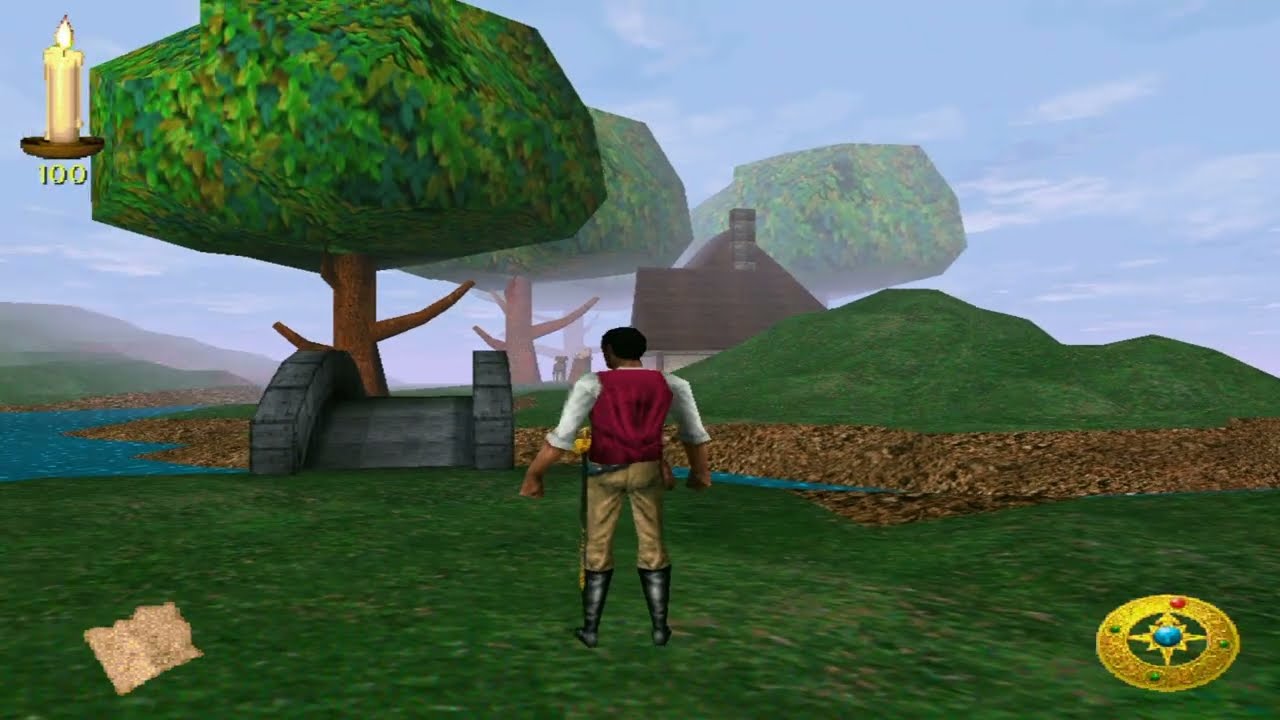In this vivid screenshot from a video game, a solitary character stands prominently at the center of an open, grassy field. He appears to be an African American man, dressed in black riding boots, tan pants, a red vest, and a white undershirt with the sleeves rolled up. A sword in a sheath is strapped to his hip. His gaze is directed towards a gray stone bridge that arches over a stream, connecting to another grassy area. Across the bridge, the landscape features a fog-enshrouded hill where a quaint house with a brown roof and chimney sits, partially obscured by round, video game-style trees. A lone dog is visible near the house, watching the man from a distance.

The sky above is light blue, dotted with clouds, and a compass adorned with jewels is located in the bottom right corner of the image. In the bottom left corner, a fragment of a map is visible, while the top left corner shows a candle with the number "100" beneath it. Surrounding elements include tan, green, red, white, black, yellow, and orange hues, which contribute to the scene’s rich color palette. The overall composition and the inclusion of interface elements like the compass, map, and candle indicate that this is indeed a screenshot lifted directly from a gameplay session.